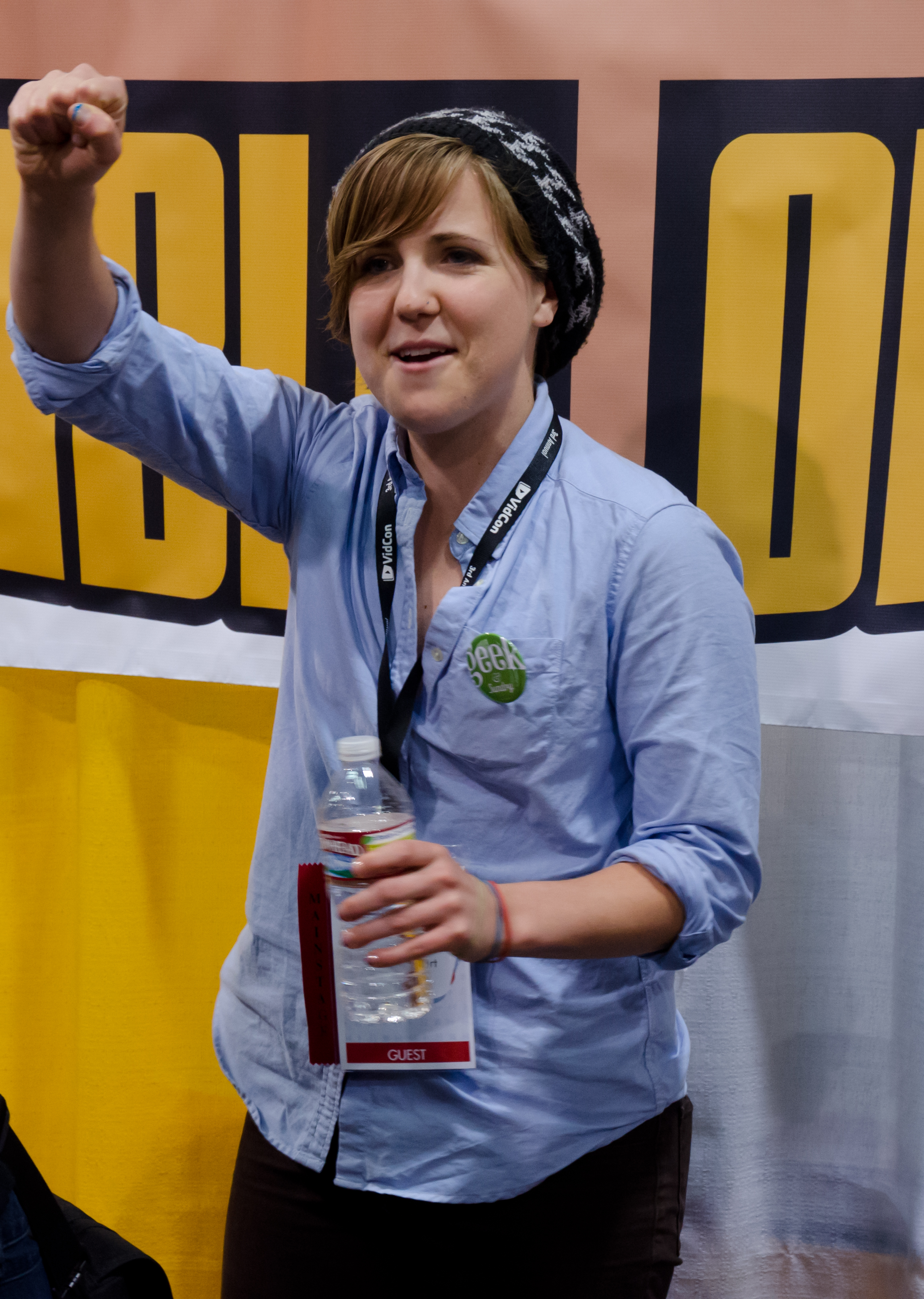This photograph features a young Caucasian woman in her mid to late 20s with reddish-brown hair, parted on the left side and swept over her forehead. She is wearing a black and gray knit beanie, which droops slightly. Her outfit comprises a light blue, button-down, open-collared shirt with rolled-up sleeves and black jeans or pants. 

Around her neck hangs a black lanyard with white lettering, ending in a white name tag that reads "guest," although the name tag is partially obscured by a water bottle she is holding in her left hand. She also has rubber bands on her wrists. On her shirt is a pin that says "geek."

The woman is smiling and facing the camera at a slight three-quarter angle, looking to the left. Her right arm is raised with her forearm bent and a fist made at shoulder height. Her left arm is bent at the elbow as she holds the water bottle in front of her waist.

She stands in front of a wall featuring a gradient background that transitions from an orangish color to gold on the left and white on the right. A banner with a black background and bold gold letters, which are unreadable due to being partially cut off and obscured by her stance, stretches across the wall behind her.